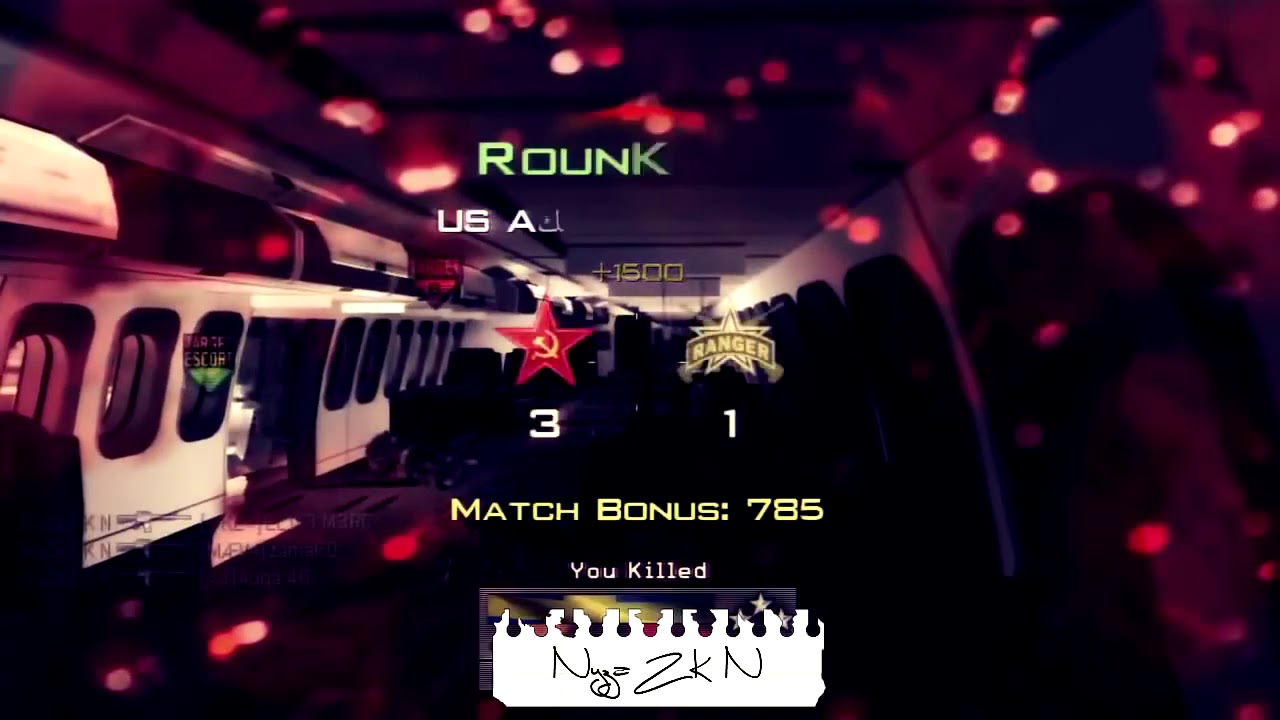This image is a screenshot from a video game, likely a first-person shooter such as Call of Duty. The scene appears to be from the end of a match, with a scoreboard indicating the Soviet Union team (identified by the hammer and sickle logo) won 3-1 against the Ranger team. In the background, there is a 3D rendered environment that could be a subway or airplane interior, though it's somewhat blurred and dark. Dramatic lighting and visible sparks add to the ambiance. The on-screen text includes "Match Bonus 785" in yellow, "You killed" followed by a handwritten note, and "plus 1500" points. There is also a stuttering text "round K" fading in, and the label "USA" with letters spaced apart. Red circles and gun icons associated with player names are visible, enhancing the resemblance to Call of Duty's UI.